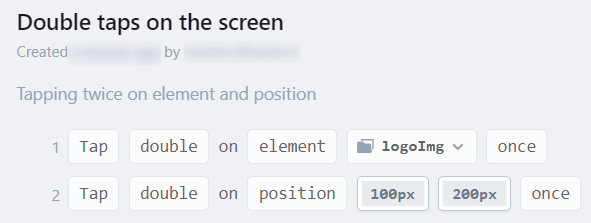The image showcases a settings window related to coding, presented in a rectangular, landscape-oriented box. The background of the window is a very light gray. 

At the top left corner, the text "Double Taps on the Screen" is displayed in prominent, bold lettering. Below this header, in smaller gray text, it states "Created by [Blurred Out]," indicating that the creator's name is obscured.

Further down, still in gray text, there is an explanatory line that reads "Tapping twice on element and position." Following this are two enumerated options, each housed within neat white boxes that suggest interactive elements such as input fields or drop-down menus.

1. The first option includes the term "Tap" followed by a white box labeled "double on element." Adjacent to this, there's another white box with a drop-down menu option displayed as "logo image," finishing with the word "once" in a third white box.
2. The second option reads "Tap double on position," and includes specific coordinates "100 px, 200 px," ending with "once," all contained within their respective white boxes.

Each detail in the image is clearly delineated, offering a structured and user-friendly interface for configuring double tap actions on screen elements and positions.